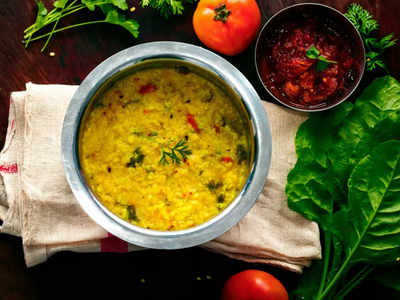This overhead image showcases a culinary spread on a dark wooden table, centered by a silver bowl with a thick rim, reminiscent of a dog bowl. The bowl contains a vibrant, yellow rice dish adorned with pieces of red and green peppers, and topped with a sprig of rosemary. This setup rests on a folded white kitchen towel featuring red stripes. Surrounding the main bowl are various elements: in the upper left corner, a sprig of parsley; in the top right corner, a jar of salsa also in a silver bowl with a tomato nearby. Additionally, in the lower right corner, there is a large basil leaf and a small Roma tomato, adding a burst of freshness to the scene. The image's dim lighting suggests a restaurant ambiance, enhancing the visual appeal of the well-composed presentation.